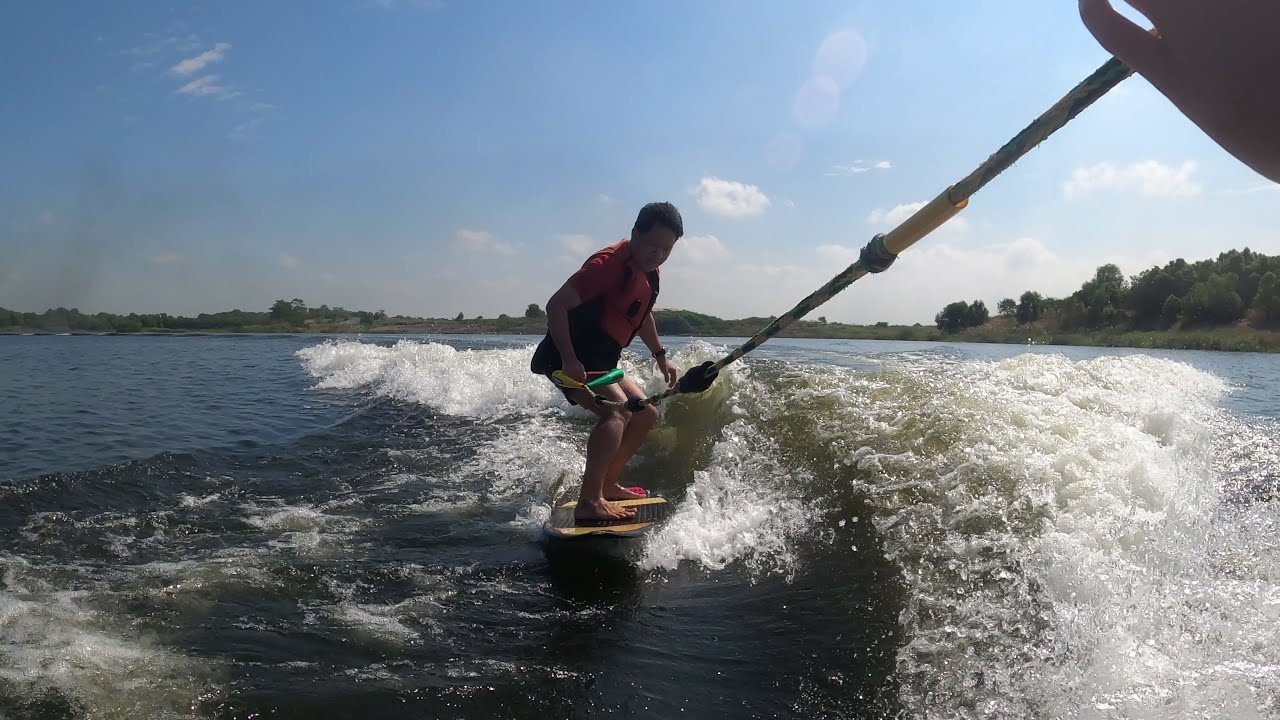A man wearing an orange life jacket, black shorts, and a short-sleeved black shirt is wakeboarding barefoot at the center of the image. He has short hair and is gripping a cable connected to a boat, visible in the upper left-hand corner of the frame. The wake from the boat creates frothy white waves around him. The surfboard he is standing on has a distinctive black and yellow color. In the distance, the shore of the lake features low rolling hills with clusters of trees, and there is an island or marsh area to the right. The water appears murky greenish-brown. The sky occupies over half of the image, painted a pale blue with some white clouds, and the left side of the image looks slightly smoky or hazy.